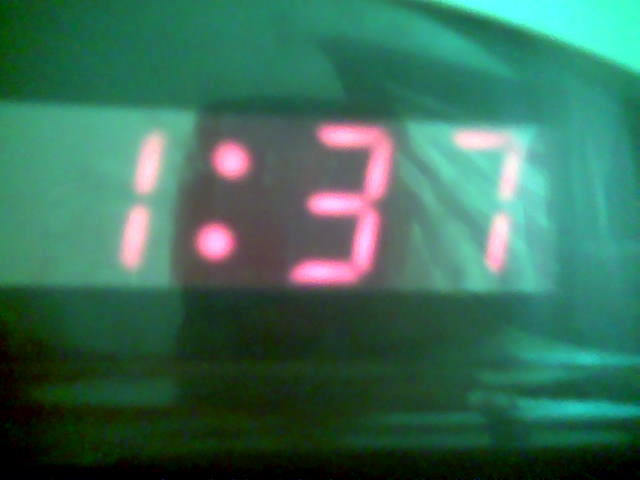This image features a digital clock face, presented in a photograph-like style that hints it could be AI-rendered. The aspect ratio is landscape, making it wider than it is tall, and the overall color tone is dominated by shades of green. The upper right-hand corner of the image displays a light teal green area, contributing to the ethereal ambiance.

Geometric shapes are visible, implying the presence of a reflective surface or a unique filter effect applied to the image. Within the composition, there is a structure resembling the contour of a dashboard or the top casing of an alarm clock. Dominating the center is an LED screen displaying the time "1:37" in glowing pink numerals, although the digits ":' and "3" are partially obscured by shadows. 

As the viewer's gaze moves downward, the image becomes progressively darker, culminating in a completely black line that spans the bottom edge of the image. The entire scene is slightly out of focus, making it difficult to discern specific details in the background, while the clock numbers remain the only clear elements in the frame.